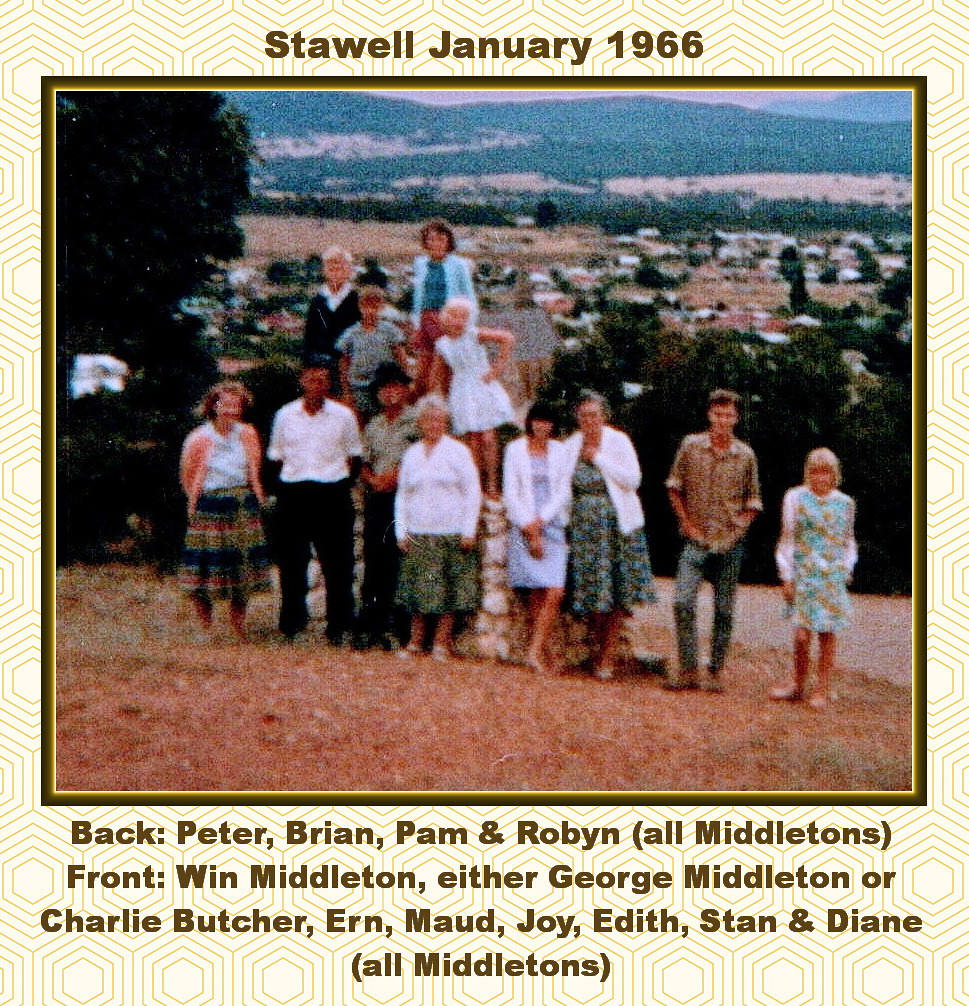In this vintage photograph, dated January 1966 and captioned "Stalwell," the Middleton family is gathered on a hill overlooking a quaint town in the background. The image captures a multi-generational family moment, with eight adults standing in the foreground, their faces reflecting a sense of togetherness and joy. Above them, four children are perched on a rock, adding a playful and dynamic element to the scene. The photograph's bottom section provides a detailed naming of all family members, further emphasizing the size and unity of the Middleton family. This evocative image beautifully encapsulates a moment in time, portraying familial bonds against the serene backdrop of Stalwell.